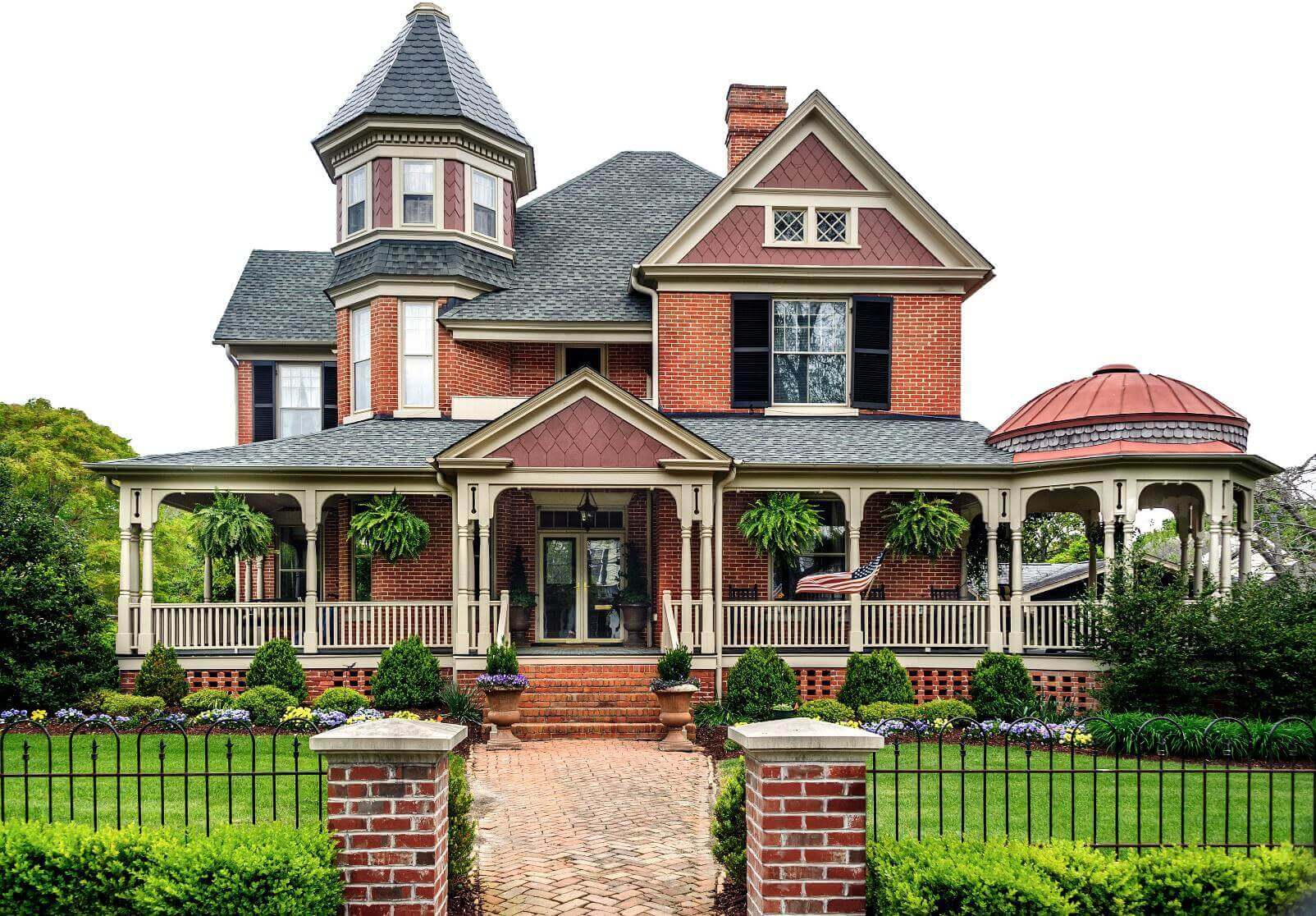This photograph captures a grand, historically-styled, brick mansion exuding an air of opulence and meticulous upkeep. Constructed primarily of red brick, the house prominently features a significant, historic brick chimney, likely increasing its market value due to the labor-intensive nature of brickwork. The Victorian architecture, reminiscent of the 1920s, includes a wraparound porch with beige moldings and supported by classic Victorian posts. The porch not only enhances the house's charm but also functions as an open gazebo area with a round, red-tiled domed roof on the right, and features Boston ferns hanging from the eaves.

The entryway is marked by a pair of stone-topped brick pillars linked by a wrought iron gate, leading to a red tile-paved walkway framed by lush, green manicured hedges. The front porch has five steps leading up to it, with a double glass front door. Adding to the stately appearance, the house includes a peaked gable above the porch entry, a steep gabled window with black shutters on the second story to the right, and a mansard-style roof behind the main gable. To the left, a rounded turret with white-cased tall windows, capped with a turreted roof, further accentuates the building’s sophisticated design.

The grounds are equally well-maintained, featuring a variety of small green shrubs, lavender, and yellow flowers, indicative of careful landscaping. The expansive lawn is lush and green, harmonizing with the detailed brickwork and architectural elegance of the house, conveying a sense of grandeur and historic preservation alongside modern upgrades.